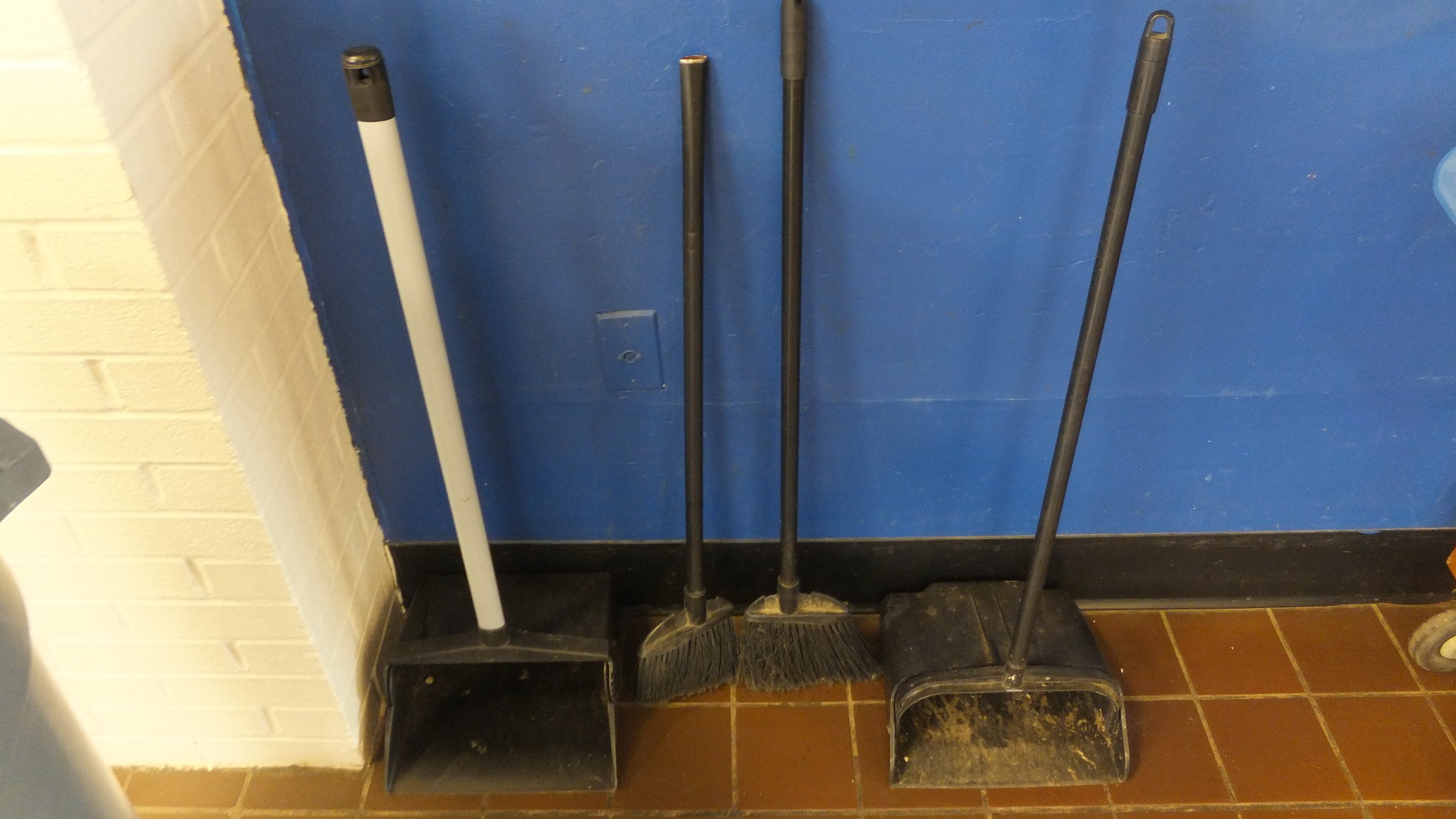In a small janitor's closet featuring a blue wall transitioning into a white brick wall, there's an arrangement of cleaning supplies on a red brick floor. The setup includes two dustpans with long handles for easy sweeping without bending down. The first dustpan, positioned on the left, has a white handle with a black top and a black plastic square bottom. Adjacent to it is a small broom with tiny black bristles and a matching black handle. Continuing right, there’s another similar broom and a second dustpan with an entirely black handle. The cluster also includes a gray trash can, an electric plug in the wall, and a glimpse of a mop. Scattered around are other essentials, including a little wheel on the right-hand side. The terracotta tiles further complement the orderly arrangement of this well-equipped closet.